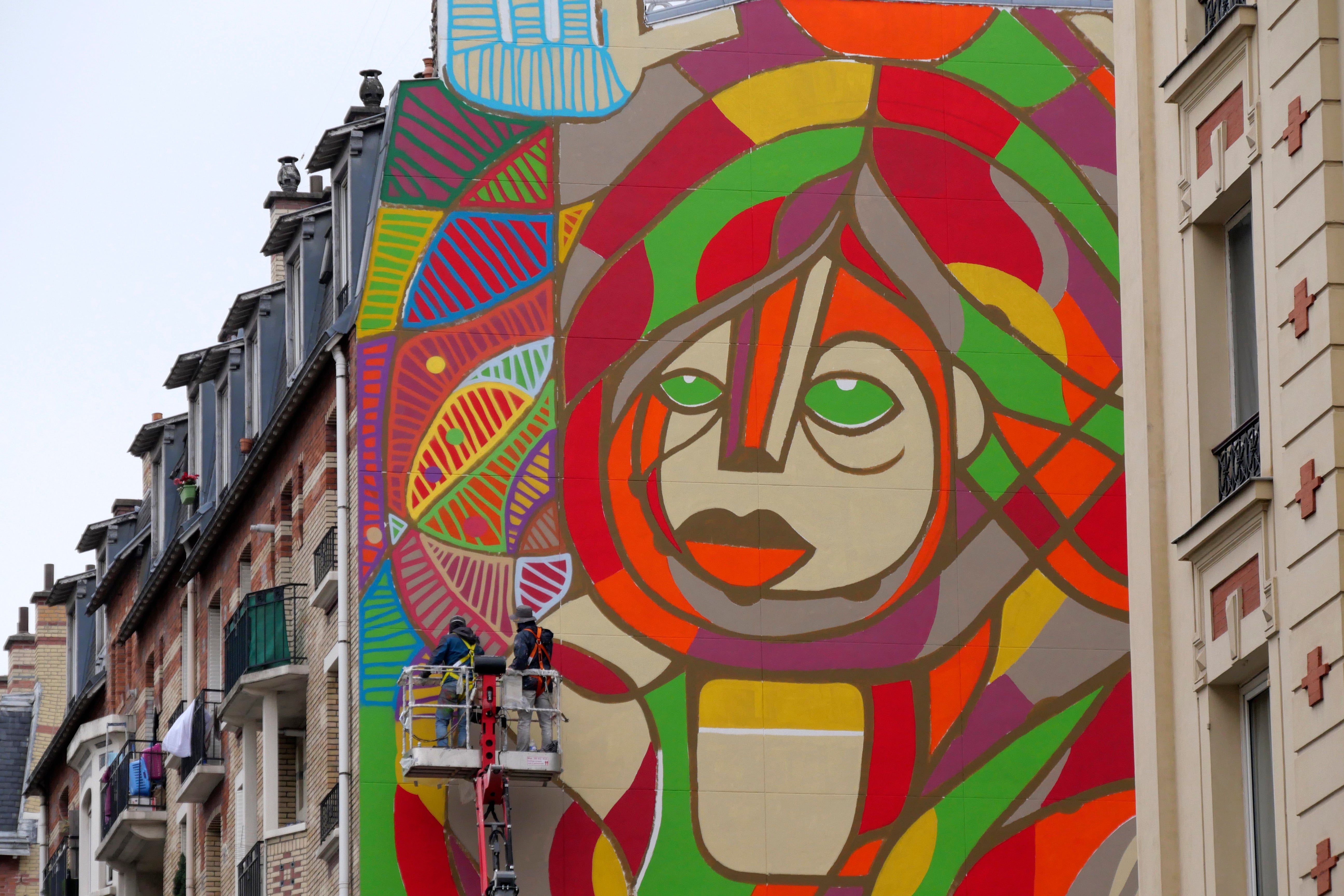The image features a colossal mural on the side of a tall, multi-story building that dominates the scene. The mural, vividly abstract in nature, portrays the ambiguous face of a female figure with piercing green eyes and white pupils, red lips, and a face that merges into a swirl of vibrant colors such as orange, red, burgundy, and yellow, creating an intricate pattern of shapes without a definitive form. Her neck is suggested through a square of yellow and beige. Above the swirls of color, part of a beige-colored hand with a light blue trim peeks through the top section of the mural.

In front of this giant artwork, two men are seen on a white lift, which is likely attached to a truck, adding the finishing touches to the mural. The lift is positioned on the left side of the mural, where only a few small sections remain to be completed.

Adjacent to the mural on the left are several townhomes, characterized by their grayish-topped chimneys and closely-built structure, leaving no space in between. Balconies adorned with various personal items, such as clothing and bedding, add a touch of everyday life to the urban setting. Each building shows off diverse elements with colors ranging from green to white, and a mix of beige and brown around the windows.

On the right side of the mural, another multi-story building with three visible floors features a beige facade with brown accent details, contributing to the densely packed, urban landscape that forms the backdrop to this vibrant street artwork.